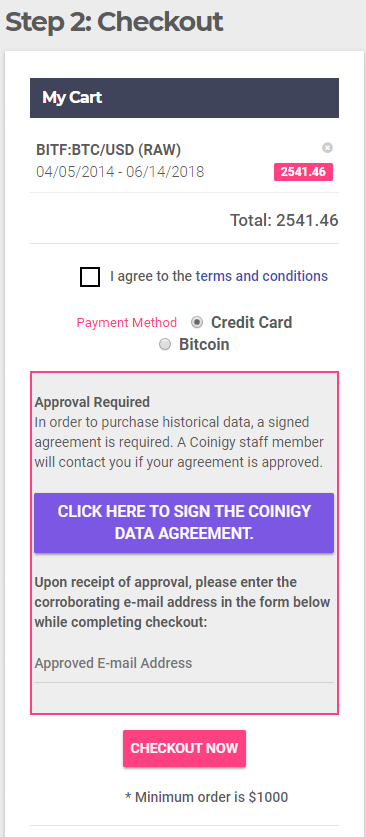This screenshot captures the checkout process of a website as viewed on a mobile phone. 

At the top, there is a grey navigation bar with darker grey text that reads "Step 2: Checkout". Below, the main section of the white page begins with a black rectangular header featuring white text that says "My Cart". 

The cart contents are detailed just beneath this header. Listed is an item labeled "BitF: BTC/USD (Raw)" with the date range "04/05/2014 - 06/14/2018". To the right of this item, in a small red rectangle, the price of "2541.46" is displayed. 

A grey dividing line separates the item details from the total price, which is listed as "Total: 2541.46". Another grey line follows, below which there is a small icon of a cube with the text "I agree to the terms and conditions" beside it. The phrase "terms and conditions" is clickable and highlighted in blue.

Underneath this, in red font, the text "Payment Method" appears, accompanied by two selections: "Credit Card" and "Bitcoin". The credit card option is currently selected. Finally, at the bottom of the screenshot, it states "Approval Required".